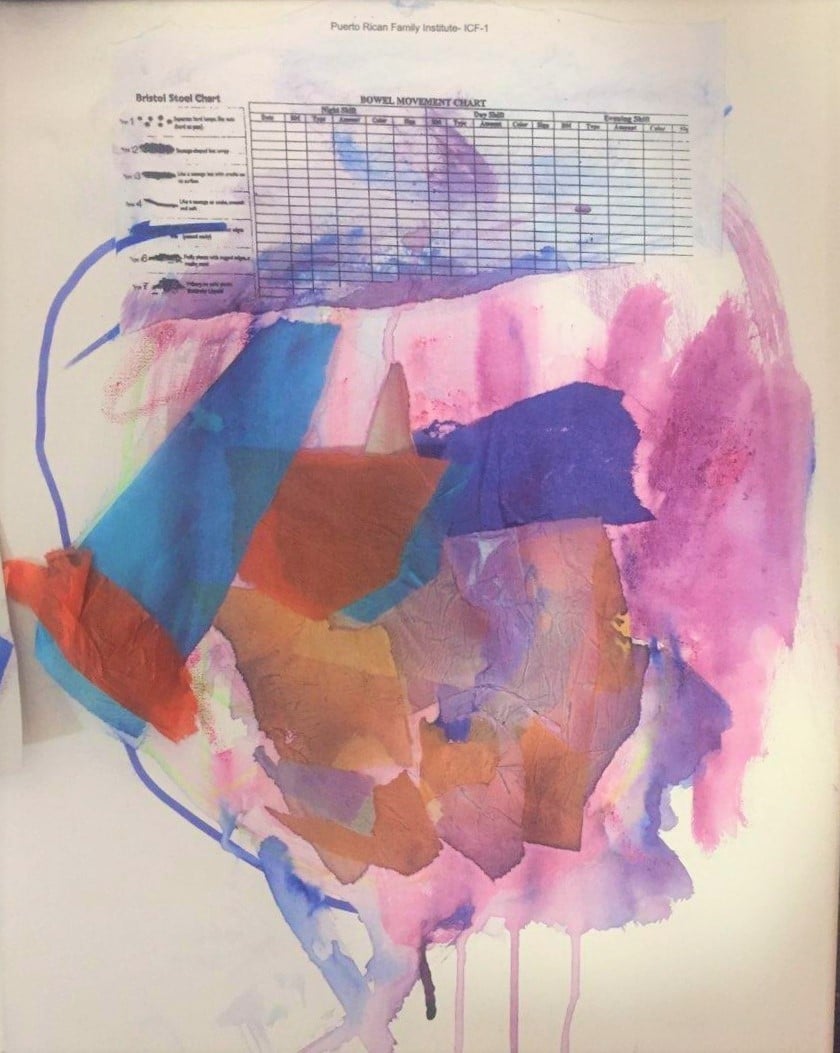This image is an abstract, collage-style illustration with a distinctly homemade feel, blending painting and scrapbooking techniques. The background features a wash of vibrant watercolors in shades of pink, purple, and blue, suggestive of fluid brush strokes running together, as if the painting was propped up to allow the colors to drip. Layered over this wash are torn shreds of tissue paper in a spectrum of hues including red, orange, blue, purple, and yellow, adding texture and depth to the composition. 

A striking element pasted atop this colorful backdrop is a piece of paper that resembles a torn and scrapped Bristol stool chart. The chart, illustrated with black rows, grids, and informative text, subtly peeks through the layers of paint and tissue paper. The title "Bowel Movement Chart" and "Bristol Stool Chart" are discernible, though somewhat obscured by the splash of colors. Notably, the artwork contains an inscription "Puerto Rican Family Institute ICF-1" at the top, further adding to its eclectic charm. The overall effect is one of vibrant, chaotic beauty, evoking a sense of spontaneity and creative freedom, akin to a piece crafted by a young child or an untrained artist.